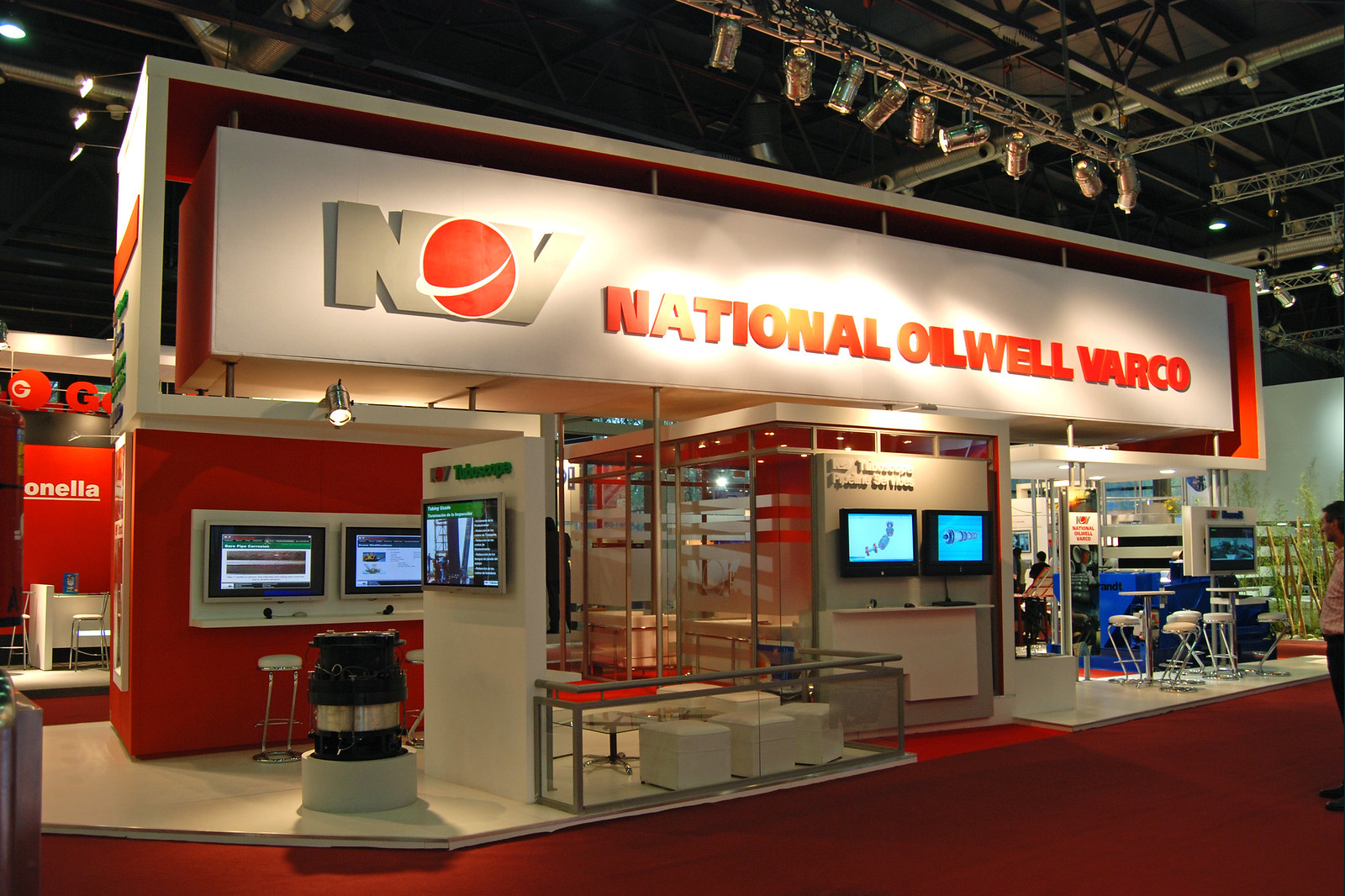This color photograph showcases a meticulously designed booth for National Oil Well Varco (NOV) inside a spacious convention hall, characterized by its industrial structure with canned lights hanging from metal frameworks. Central to the image is NOV's prominent display area, adorned with their stylized orange and white logo, where the “O” resembles an orange planet. The booth itself is an elaborate setup within the larger convention space, featuring sleek, modern furniture including small stools and square cushion seats, arranged around tiny glass tables and several computer monitors mounted on walls. The entire area is dominated by bright orange and white panels, giving it a cohesive and vibrant appearance. Behind the NOV display, there's another booth marked "Onella," similarly styled in orange and white. A partially visible man stands at the bottom right of the photo, seemingly inspecting or setting up the display, suggesting a preparation phase or a moment during a quieter time in the convention.